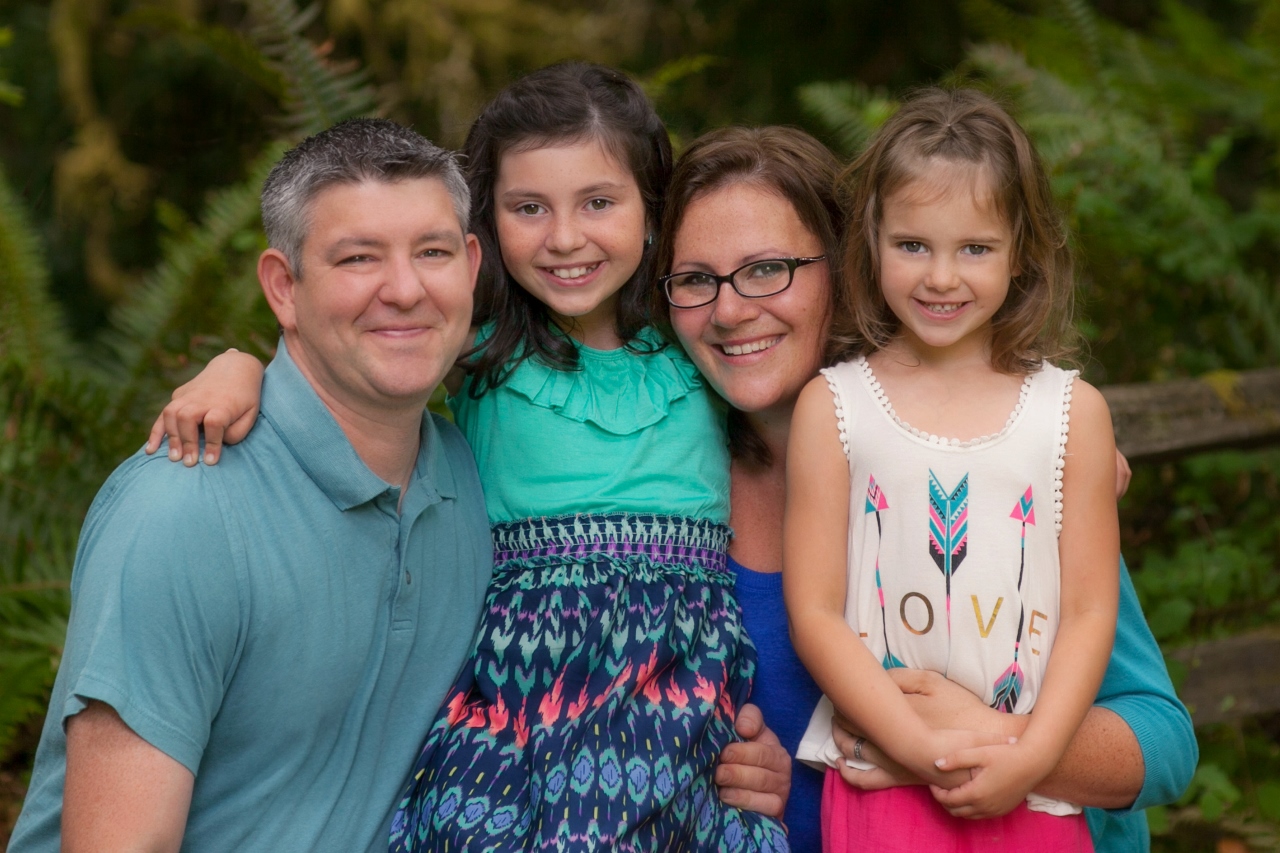In the image, from left to right, there are two adults and two young girls:

The father stands first, with graying hair that is black on top and gray on the sides. He is clean-shaven and wears a short-sleeved turquoise polo shirt. 

Next to him is the older daughter. She has long, brown hair and is dressed in a green top paired with a colorful, possibly batik-patterned skirt. The skirt has stripes in blue, pink, green, and light blue.

To her right is the mother, who also has long brown hair and is wearing black-rimmed glasses. She is dressed in what appears to be a royal blue top or dress. There is some confusion as her arm, wrapped around the youngest daughter, seems to show a turquoise sleeve, suggesting she might be wearing a cardigan that isn't visible from the front.

Finally, the youngest daughter is pictured with shoulder-length brown hair. She wears a sleeveless top adorned with the word “love” and three multicolored arrows—two pointing up and one pointing down. She is dressed in pink, 'Barbie-pink' pants or a skirt with a fern or foliage pattern.